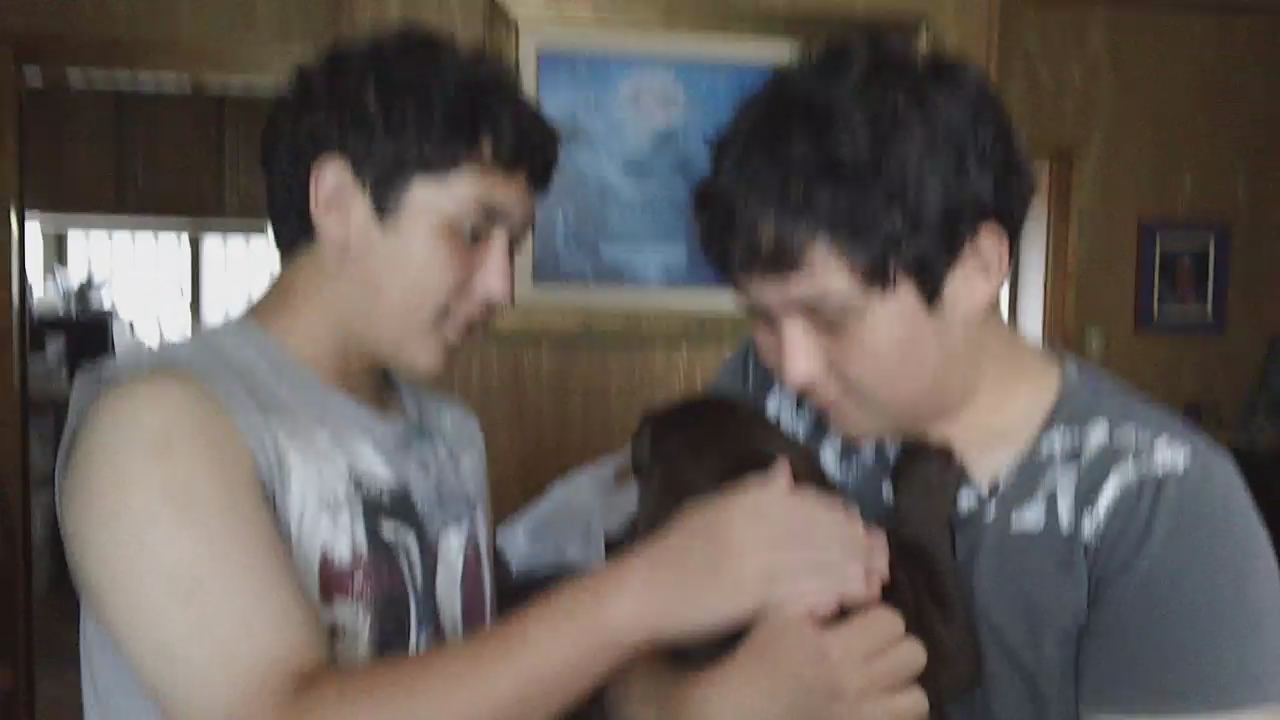The image is a very blurry, color photo capturing two boys who seem to be brothers or close relatives. They are positioned mid-chest up, both with dark, somewhat curly hair. The boy on the right, wearing a gray t-shirt with white print across the shoulders, is holding a small, black or brown puppy in his right arm. He is looking down at the puppy. The boy on the left, slightly older and chubbier, has a sleeveless gray tank top featuring a graphic print on the front. He is reaching out with his right hand to pet the puppy. In the background, the room has wood-paneled walls adorned with framed artwork, including a painting with a blue hue and a light brown frame. Light streams in from a window with pulled-up slat blinds on the top left, just above the older boy's head. Though the image is extremely out of focus, these details are faintly discernible.